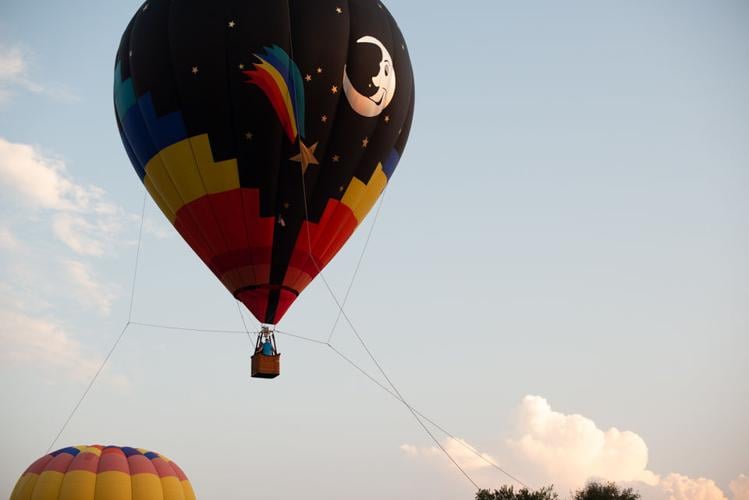This landscape photograph captures a vivid scene of two hot air balloons against a serene, light blue sky scattered with white, fleece-like cumulus clouds, predominantly on the left side. In the foreground, slightly off-center to the left, a striking hot air balloon takes center stage. This balloon is primarily dark blue, adorned with a celestial theme featuring stars and a white crescent moon with a face. A gold shooting star with a tail of blue, yellow, and red adds a touch of magic. The balloon's lower section showcases stripes of aqua, blue, yellow, and red, leading down to a small basket where two figures stand, secured by ropes anchoring the balloon to the ground. In the bottom left corner, the top of another hot air balloon is visible, predominantly yellow with sections of red, blue, and an orangey-brown color, adding more vibrant hues to the image. The bottom right corner reveals the tips of green trees, completing this enchanting and colorful outdoor scene.